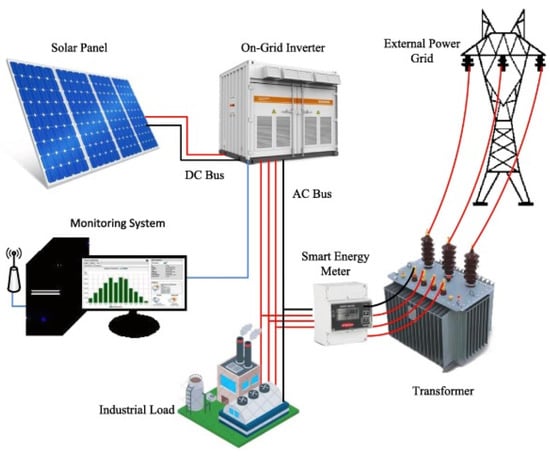The image depicts a detailed labeled diagram of a solar energy system on a white background, organized in a clockwise direction from the center. Starting from the upper left corner, the diagram shows a blue solar panel divided into four panels labeled "Solar Panel." Connected to the solar panel are red and black wires marked "DC Bus" that link to a white box labeled "On-Grid Inverter." From the inverter, three red lines and one black line emerge, labeled "AC Bus," and lead downwards to a section labeled "Industrial Load," which depicts a factory-like structure. 

In parallel, another set of wires branches off to the right, connecting to a white box labeled "Smart Energy Meter," which then extends to a larger gray box marked "Transformer." The transformer, characterized by its gray ridges resembling heat sinks and three central posts, is connected via three red lines to a power line structure labeled "External Power Grid." 

Additionally, a blue line extends from the inverter down to the left, connecting to a computer system labeled "Monitoring System," with a computer tower that also appears to include a router or wireless antenna. This comprehensive diagram illustrates the interconnected components of an on-grid solar power system, including the solar panel, inverter, smart energy meter, transformer, and external power grid, alongside monitoring capabilities.